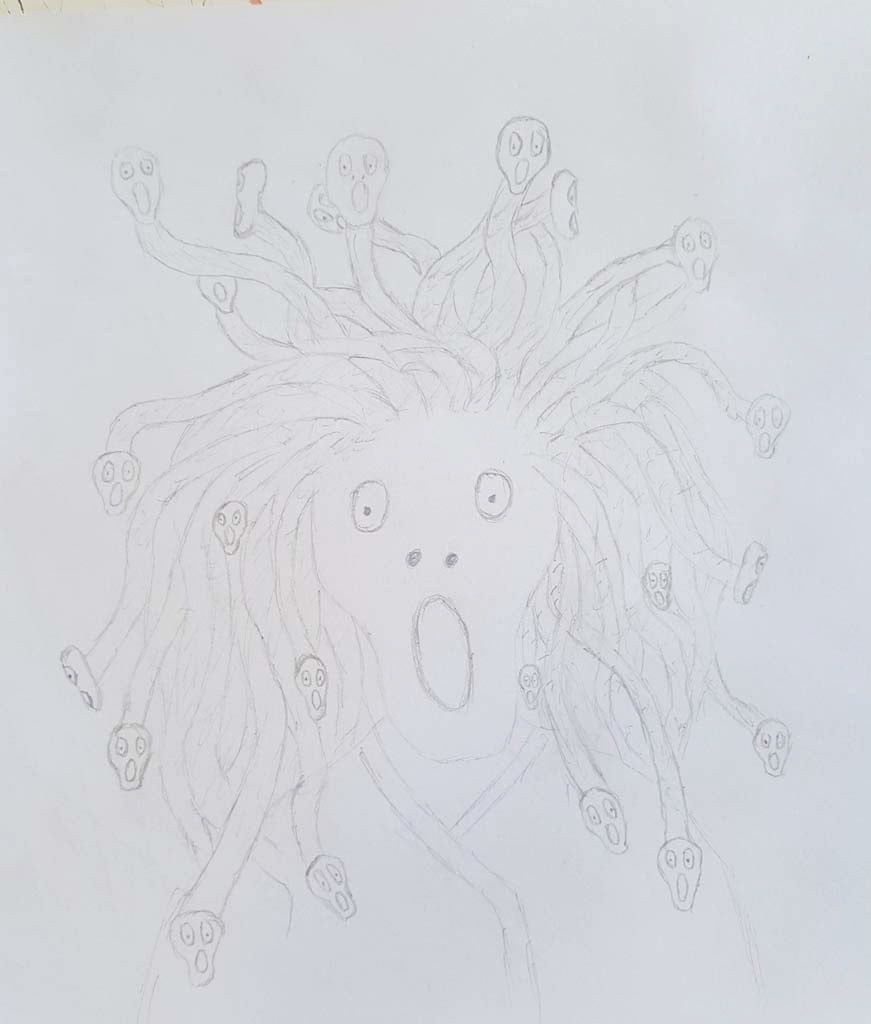This image captures a high-resolution photograph of a detailed pencil drawing on an elegant sheet of drawing paper. The paper is pristine white, devoid of any lines or markings, suggesting it is of a higher quality, possibly designed specifically for artistic purposes rather than standard construction paper.

At the heart of the drawing is a striking depiction of Medusa. Her face is the focal point, characterized by wide, expressive eyes, diminutive nostrils, and a dramatically open, round mouth. This central figure exudes a mystic and slightly eerie presence. Encircling her head are numerous locks of hair, each transforming into a likeness of her own face at the tips. These smaller faces mirror her rounded contour, with the upper part slightly wider, tapering into a rounded chin. Each miniaturized face also features similarly wide eyes and an O-shaped mouth, evoking a sense of unity and repetition within the chaos of her serpentine locks.

The intricate details of the drawing, captured on this fine piece of paper, highlight the artist’s skilled craftsmanship and imaginative interpretation of the mythical Medusa, blending elements of alien-like features with the traditional snake-haired visage.